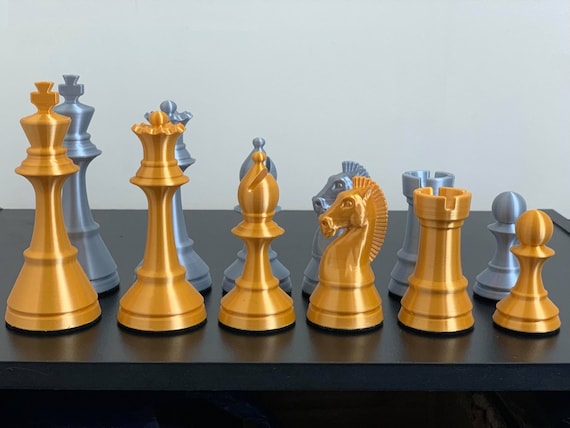The image features a meticulously arranged set of chess pieces on a glossy, dark brown wooden table. The chess pieces are organized in two rows, with the front row consisting of six gold-colored pieces and the back row comprising six silver-colored pieces. Each row presents a lineup of a king, queen, bishop, knight, rook, and pawn from left to right. The gold and silver pieces are notably shiny, with distinct light reflections enhancing their metallic hues. The gold pieces are placed directly in front of their silver counterparts, creating a mirrored effect. The wooden table surface is highly polished, allowing the pieces' reflections to be clearly visible. The side of the table is a darker shade of brown compared to the top. The background is a plain, light bluish-gray color, ensuring that the focus remains solely on the chess pieces. The overall image is well-lit and has a bright and clear setting with no additional objects or text, making the chess pieces the central focus of the photograph.